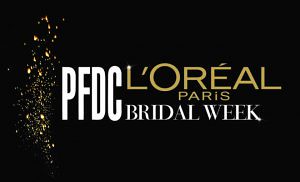The advertisement features a medium-sized black rectangular background. Along the left side, a spray of gold glitter or confetti extends almost the full height of the image, giving a dynamic, celebratory feel. Dominating the center of the black background are the large white letters "P.F.D.C." In a vertically aligned format to the right of this, "L'Oreal Paris" is written in large yellow text, with "L'Oreal" being the tallest, followed by "Paris" centered beneath it. Below "L'Oreal Paris," the words "Bridal Week" are displayed in white, capital letters. The structured typography and glitter detail create a simple yet eye-catching design, ideal for a digital advertisement on web pages.